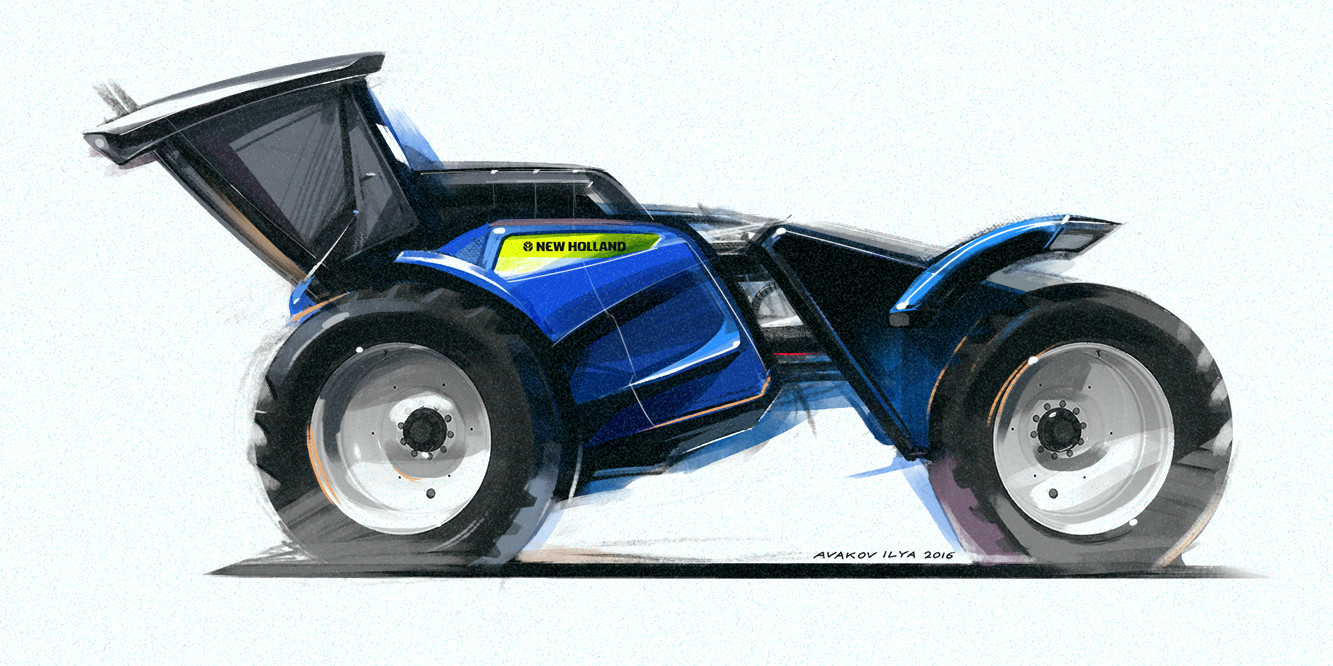This detailed artwork depicts a futuristic, large-scale model of a farming vehicle—possibly New Holland machinery—featuring striking blue painted bodywork and vibrant yellow background accentuating the "New Holland" logo. The vehicle exhibits massive black tires with distinct white-silver hubs. A small canopy, situated in the top left corner, includes a blue handle for entry and exit, indicating where a driver would sit. The vehicle's overall design shares similarities with a race car or a monster truck, evident from its large, uncovered wheels with chrome fenders positioned over the front and back wheels. Additional details such as a black roof, a small green window, and a red center light enhance the futuristic aesthetic. At the bottom of the image, the artist's signature, "AVA KOV ILYA 2016," can be seen, confirming the creation date and providing an intriguing finishing touch to the composition.